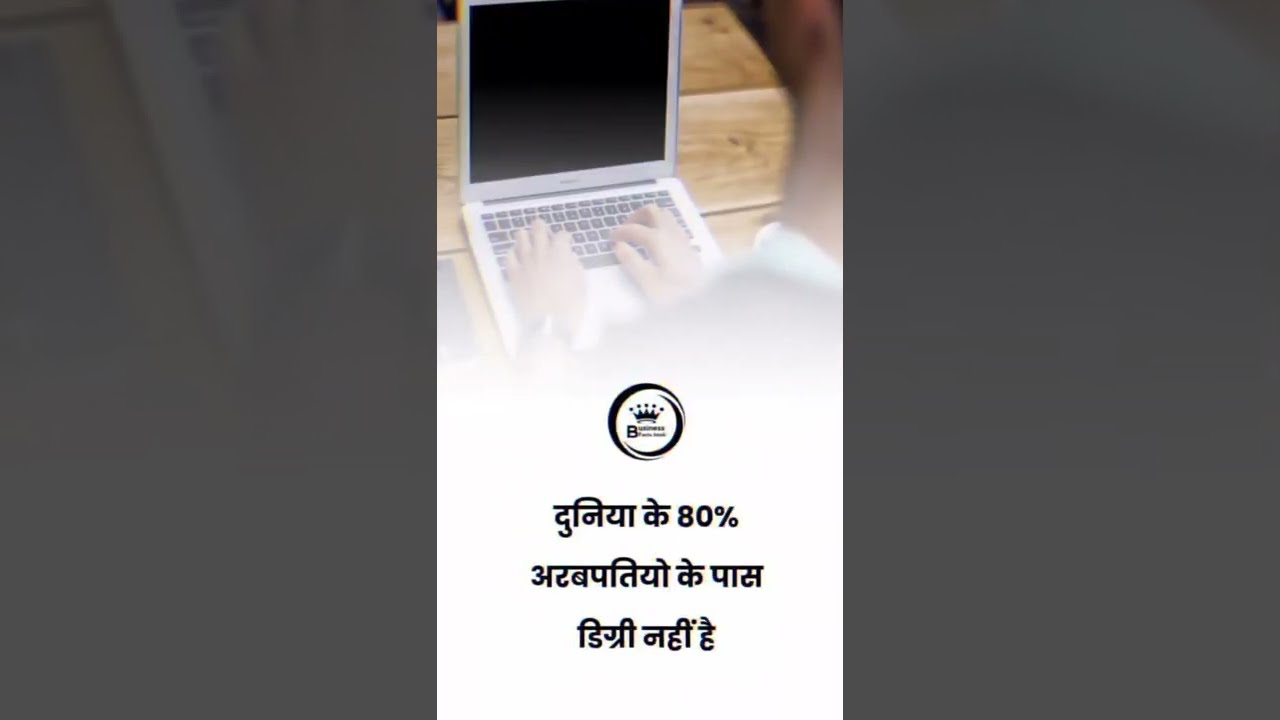The image features a vertical banner set against a predominantly blurry, grayish background, hinting at a photograph. The central focus of the banner is a young man working on a white laptop that has a black keyboard, positioned on a wooden table. The perspective is from slightly behind and to the left of the man, showing the lower left side of his head, his neck, and his hands on the keyboard. The man appears to be wearing a bracelet or wristwatch on his left wrist.

While the left and right sides of the image are dark and somewhat blend into the gray background, the central portion is vibrant and clear. The laptop in the middle of the banner has an entirely black screen with illegible text in a language that appears to be Middle Eastern, possibly Sanskrit or Hindu. About halfway down the banner, the image transitions to white, revealing a logo with a crown and the letter 'B' inside a black circle, accompanied by some small, indecipherable text. Further below, more foreign text is displayed, including a prominent "80%" in numerals.